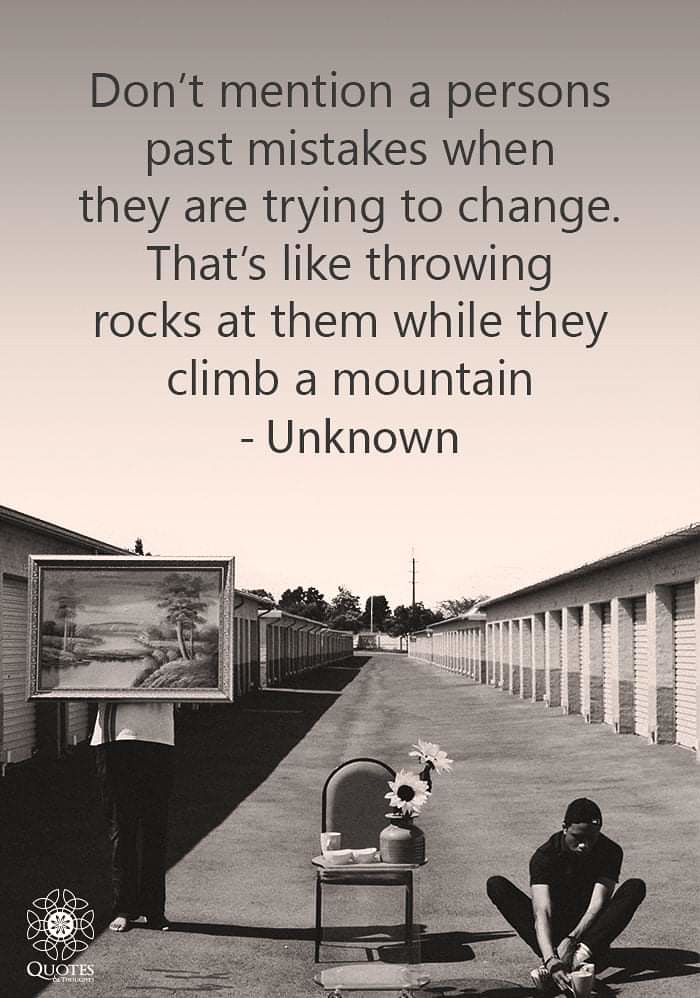The black and white poster captures a poignant scene at a storage facility, framed by rows of storage units that stretch endlessly towards a tree-lined horizon and a distant power pole. Central to the image is a young Black man, dressed in black, seated with his legs crossed and a cup in hand on the blacktop. Beside him is an intriguing arrangement: a chair adorned with a vase of large, decorative daisies, two saucers, another cup, and a serving tray on the ground beneath it. To the left of the chair stands another youth, visible from the mid-waist down, holding an ornate framed painting depicting a serene country landscape with trees and a stream. Scrawled across the top of the image in bold text is the quote, "Don't mention a person's past mistakes when they are trying to change. That's like throwing rocks at them while they climb a mountain." Signed UNKNOWN. The bottom left corner of the image features a logo with the word "quotes."